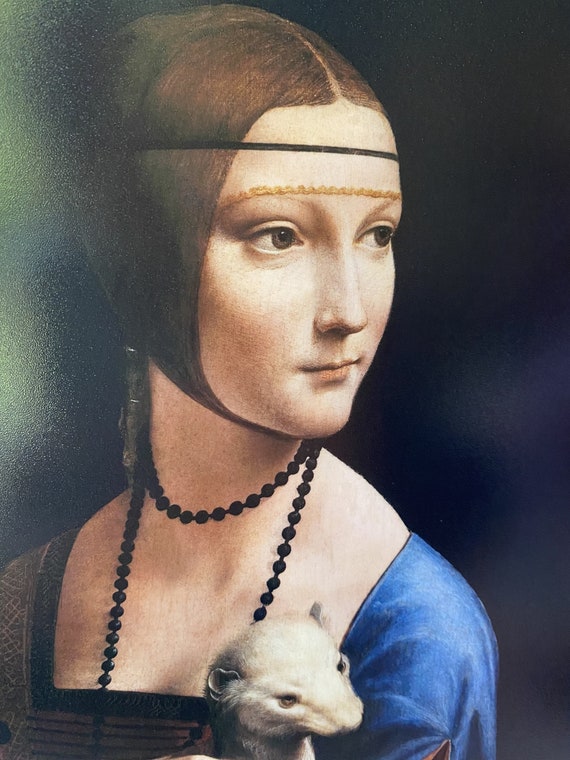This detailed illustration showcases Leonardo da Vinci's famous painting "Lady with an Ermine". The young woman, depicted from the head down to just below the shoulders, has chin-length, sleek brown hair parted in the center. She wears a thin black headband across her forehead, and a gold or yellow band just above her eyebrows. Her fair skin and brown eyes give her a gentle expression as she gazes to the right, her lips closed in a poised, unsmiling demeanor. Dressed in a blue cloak over a brown dress with darker, differently patterned sleeves partly obscured by shadow, she accessorizes with double strands of black beads around her neck. In her arms, she delicately holds a white ermine, positioned at the center bottom of the painting. The background is painted in a stark black, highlighting her serene presence in this vintage masterpiece.